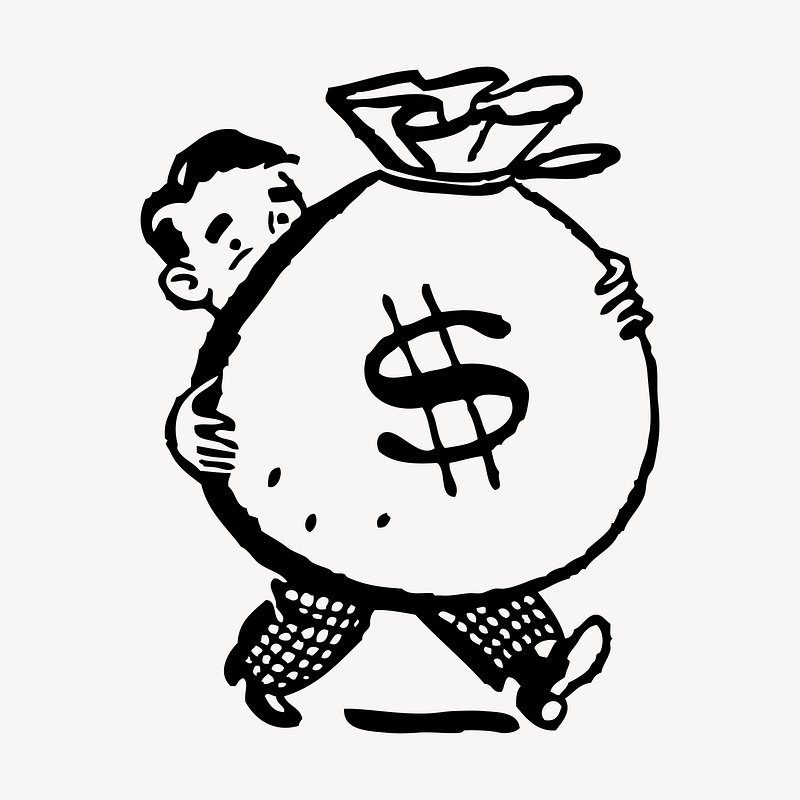This black-and-white cartoon-style illustration features a young boy with dark hair and bushy eyebrows, partially obscured by the giant money bag he is carrying. His eyes are simple circles, adding to the cartoonish feel of the drawing. The boy is dressed in patterned, black-and-white checkered pants and black dress shoes, suggesting a modest yet playful attire. The massive bag, adorned with a prominent dollar sign, dominates the scene, tied at the top with a rope and bulging out. The bag is so large that it conceals most of the boy’s body, including his thighs, with only his wide-stancing legs visible beneath it. His hands are spread wide, gripping the bag tightly as he appears to be moving forward, suggesting the weight and size of the bag relative to his small stature. The entire background is unadorned white, emphasizing the simplicity and focus on the central characters: the boy and the money bag.